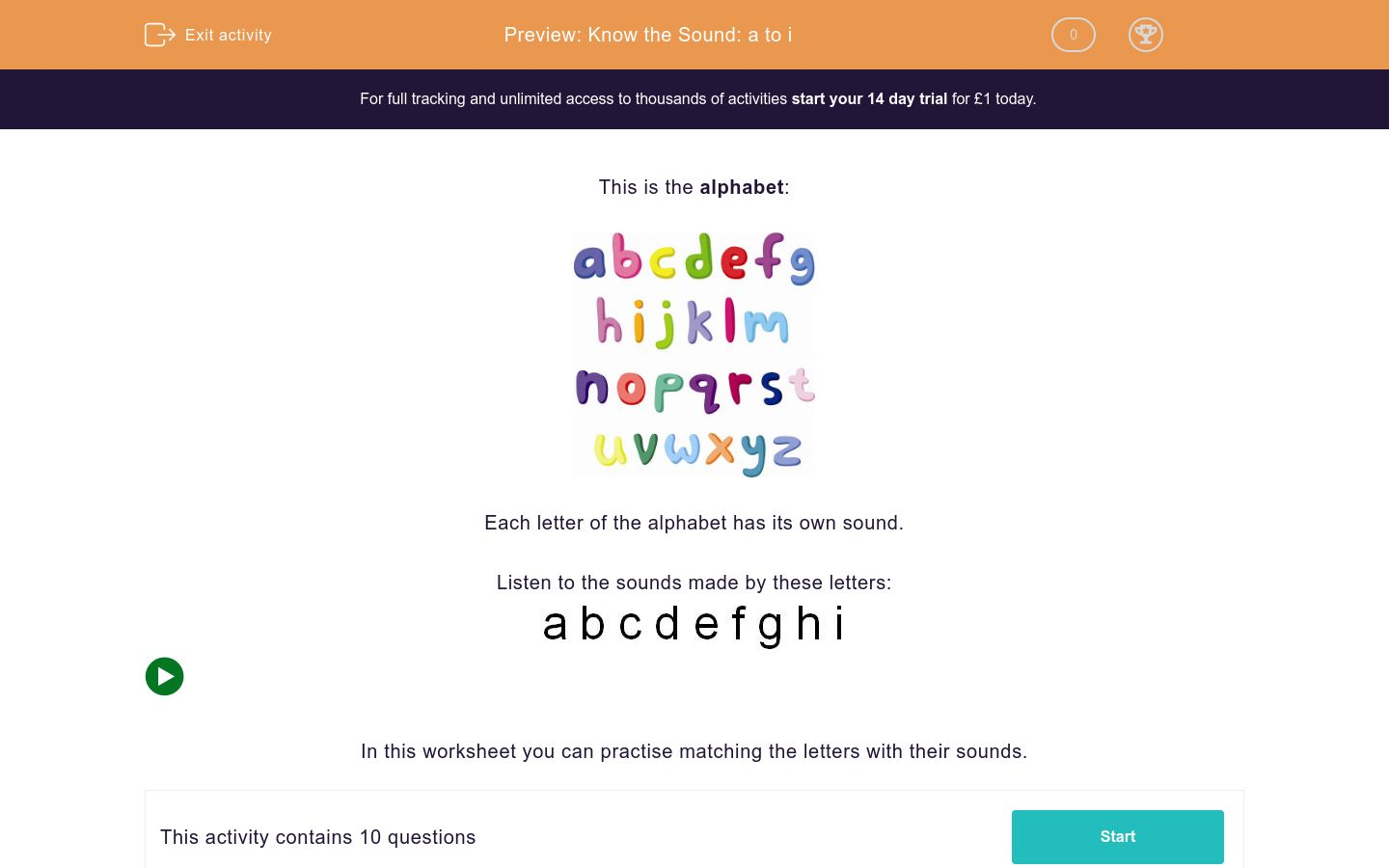Here is a polished and detailed caption for the described image:

---

At the top of the page, an orange header sets a vibrant tone. The header includes two text elements: "Preview: Know the Sounds A to I" prominently centered and "Exit Activity" on the left side. On the right side of the header, you will find the score and a leaderboard. Below the header, another text block appears on a navy background, stating, "For full tracking and unlimited access to thousands of activities, start your 14-day trial for one pound today."

The main section of the page features a white background. Centrally aligned, there is a text introducing the alphabet from A to Z. The letters are displayed in various colors: A in blue, B in pink, C in red, D in green, E in purple, F in blue, G in orange, H in yellow, and I in pink. Below this colorful alphabet, the text reads, "Each letter of the alphabet has its own sound. Listen to the sounds made by these letters: A to I."

At the bottom of the page, instructions are provided on a navy background, accompanied by a green "Play" button on the left side. The instructions declare, "In this worksheet, you can practice matching the letters with their sounds." Additionally, a note says, "This activity contains 10 questions." The bottom-right corner features a prominent green "Start" button to initiate the activity.

---

This caption effectively organizes and presents all the details found in the original description.